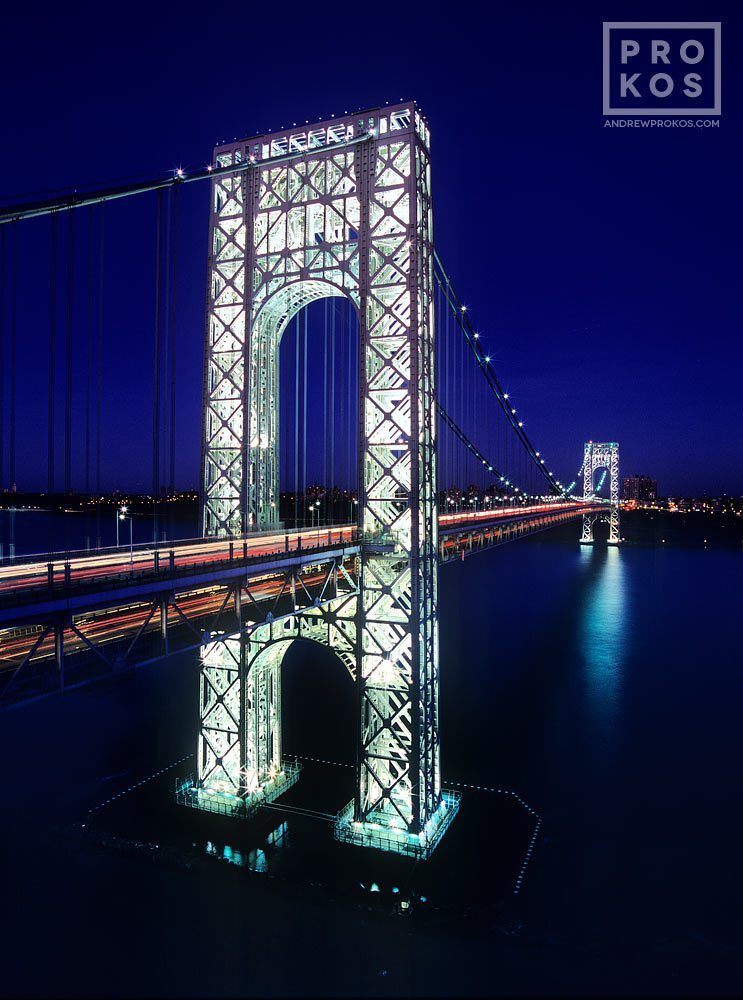In this nighttime photograph of a grand suspension arch bridge, the structure is prominently illuminated against a deep blue sky that seamlessly transitions into a darker blue river below, adding to the serene ambiance. The bridge, resembling the design of iconic structures like the Brooklyn Bridge or the Roebling Bridge in Cincinnati, features decorative crisscross supports that light up brilliantly, enhancing its architectural elegance. With an imposing tower shaped like a block letter "A," the bridge is adorned in bright white lights, while a continuous strip of orange illumination runs along its length, highlighting the sturdy, conservative style of its framework. Hanging ballasts support the structure, and you can observe traffic in motion as streaks of red taillights and white headlights blur through the scene. In the distance, small city lights twinkle, casting a gentle glow without the presence of towering skyscrapers. The bridge spans a gleaming river, adding a reflective charm to the image. At the top right corner, there's a slightly rectangular watermark box with the text "PRO" over "KOS" in capital letters, and below it, in smaller capital text, it reads "andrewprokos.com." The clear, starless sky above completes this stunning nighttime cityscape.